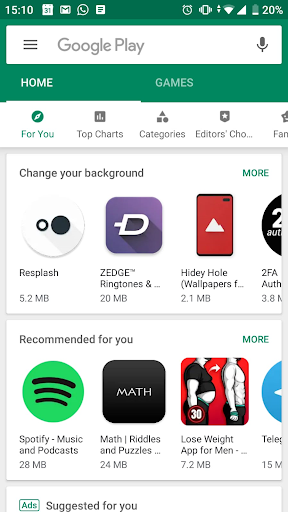In this image captured on a cell phone, we observe the Google Play Store interface. The top portion of the screen displays the phone's status bar, indicating the time, calendar icon, mail icon, an active alarm, Wi-Fi signal strength, network signal, and battery level. Below the status bar, the interface is dominated by a green header that transitions into a white search bar containing the words "Google Play," confirming that this is indeed the Google Play Store app.

Beneath the search bar, navigation options feature prominently, including buttons for "Home" and "Games," with the "Home" button currently selected. Further options include tabs for "For You," "Top Charts," "Categories," and "Editor's Choice."

As we move down, a section showcasing various wallpapers appears, including icons for "Change Your Background" with associated choices such as ResSplash, Zedge, and Hidey Hole Wallpapers. Below this, the image highlights a "Recommended for You" segment displaying app icons for popular applications and utilities like Spotify, Math, and a weight loss app.